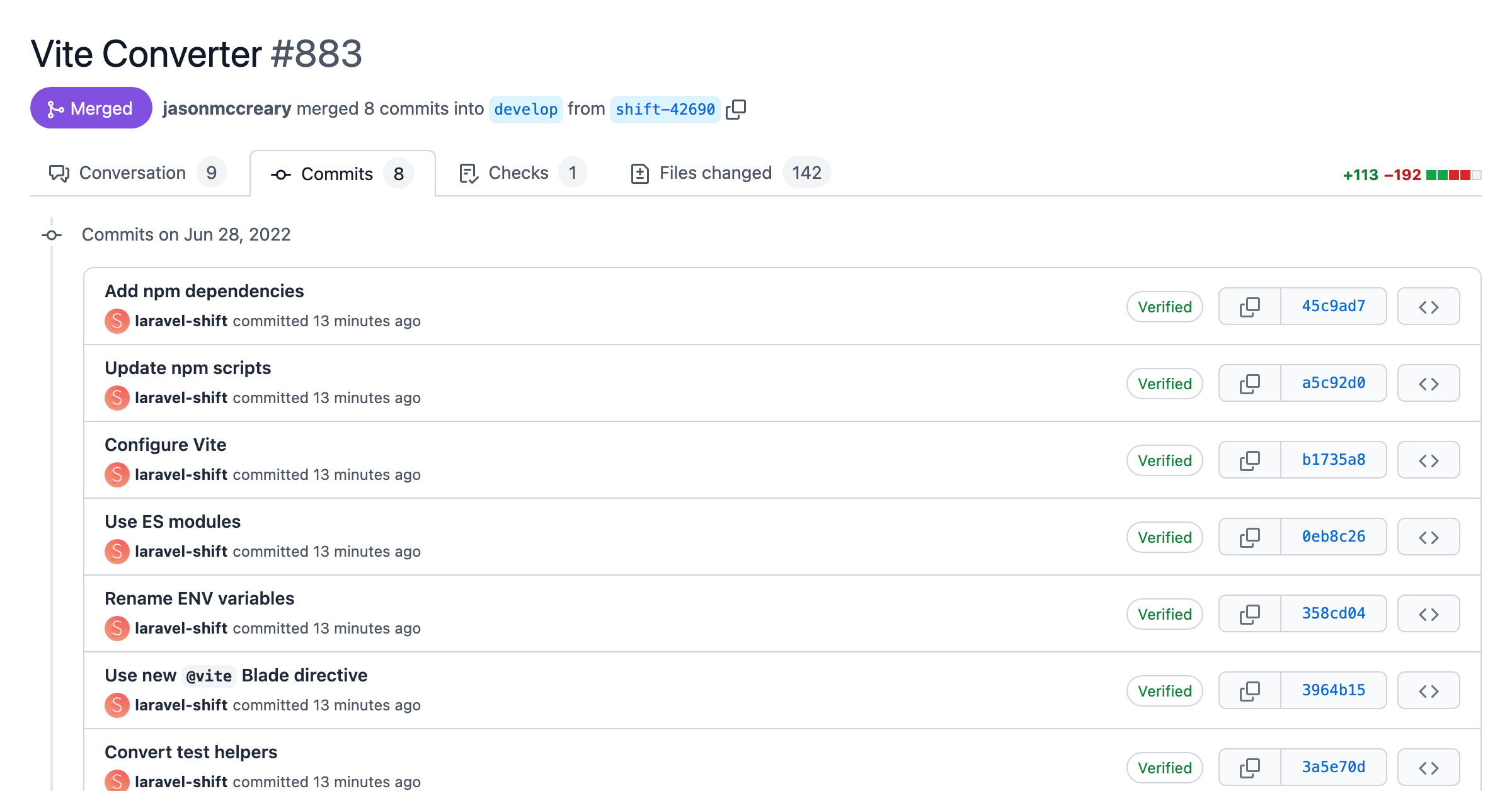Here is a cleaned-up and detailed caption for the given image description:

---

This image is a screenshot taken from a laptop, displaying a web interface in landscape mode. In the upper left-hand corner, it shows "Vite Converter #883." Following this, there is a purple button labeled "Merge" with white text, adjacent to a share icon. 

Next to these elements is the bold text "Jason McCreery," indicating the name of the individual. The text further reads "merged 8 commits into blue-develop from blue-shift-42690," with a copy icon beside it.

The subsequent row contains several tabs labeled as follows: "Conversation (9)", "Commits (8)", "Checks (1)", and "Files Changed (142)". At the end of this row, numerical changes are indicated with a "+113 -" denoting 113 additions and "-192" representing 192 deletions, accompanied by green and red squares.

The focused tab is the "Commits" tab, the second in the sequence. Listed under "Commits," various actions and timestamps are detailed:

1. **June 28, 2022:** 
   - **Add NPM dependencies:** Committed 13 minutes ago by Laravel Shift.
   - **Update NPM scripts:** Committed 13 minutes ago by Laravel Shift.
   - **Configure Vite, use ESM modules, rename ENV variables, use new @vite blade directive, convert test helpers.**

Each commit entry on the right features a "Verified" button and a "Copy" icon. The commits are identified by unique codes:
- The top commit code is **45c9ad7**.
- The bottom commit code displayed in blue is **3a5e7od**.

---

This caption offers a comprehensive and organized description of the screenshot, highlighting pertinent details for clarity.